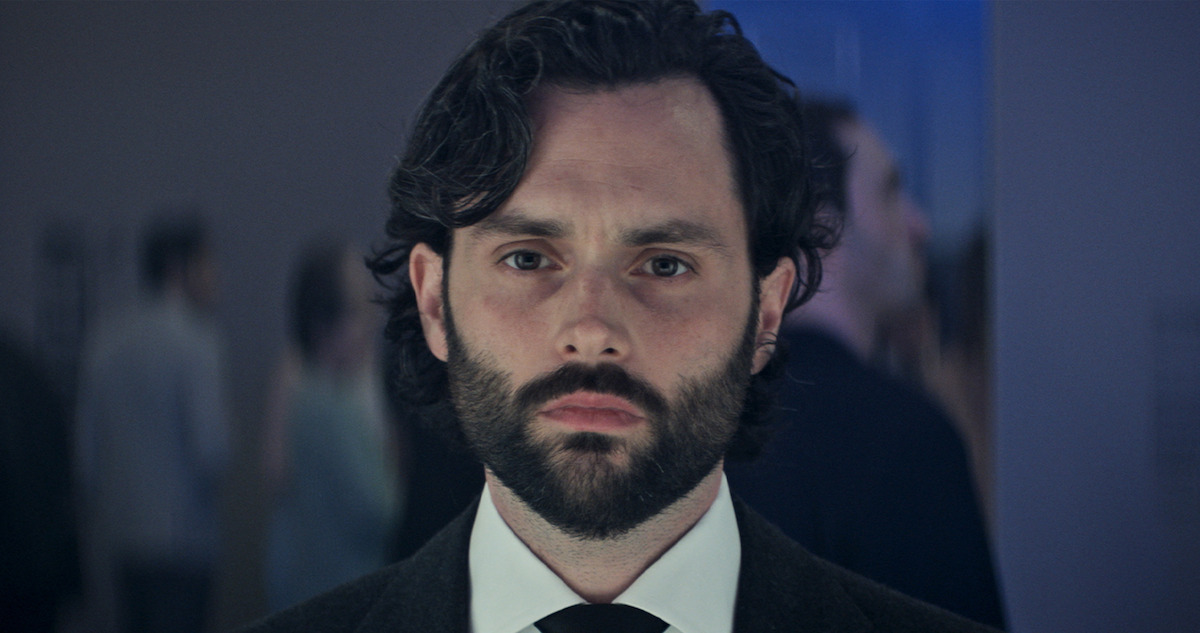This detailed photograph features Penn Badgley, evidently from the TV show "You," displaying a cinematic quality with its dim lighting and soft focus shading. Positioned front and center, the image captures Penn's head and shoulders, emphasizing his composed, deadpan expression. He appears to be in his late 20s to early 30s, sporting dark, wavy hair that reaches the nape of his neck and is side-swept, revealing slight thinning at the part. His facial features include thick bushy eyebrows, a small pudgy nose, and dark brown eyes. Penn is adorned in a formal outfit: a white collared shirt, a black tie (cut off at the bottom of the image), and a black suit jacket. His beard and mustache are full, with a hint of five o'clock shadow visible on his neck beneath the beard.

The backdrop is a blurred, bokeh effect in muted blues and grays, highlighting Penn as the sharply focused subject. The background hints at a cocktail party setting, with at least three indistinct figures—one in a suit and another in a dress—fading softly into the dim lights and shadowy hues. The overall composition conveys an intriguing mix of clarity and mystery, with Penn Badgley's expression and the softly lit, out-of-focus environment evoking a still from a dramatic moment in the series.